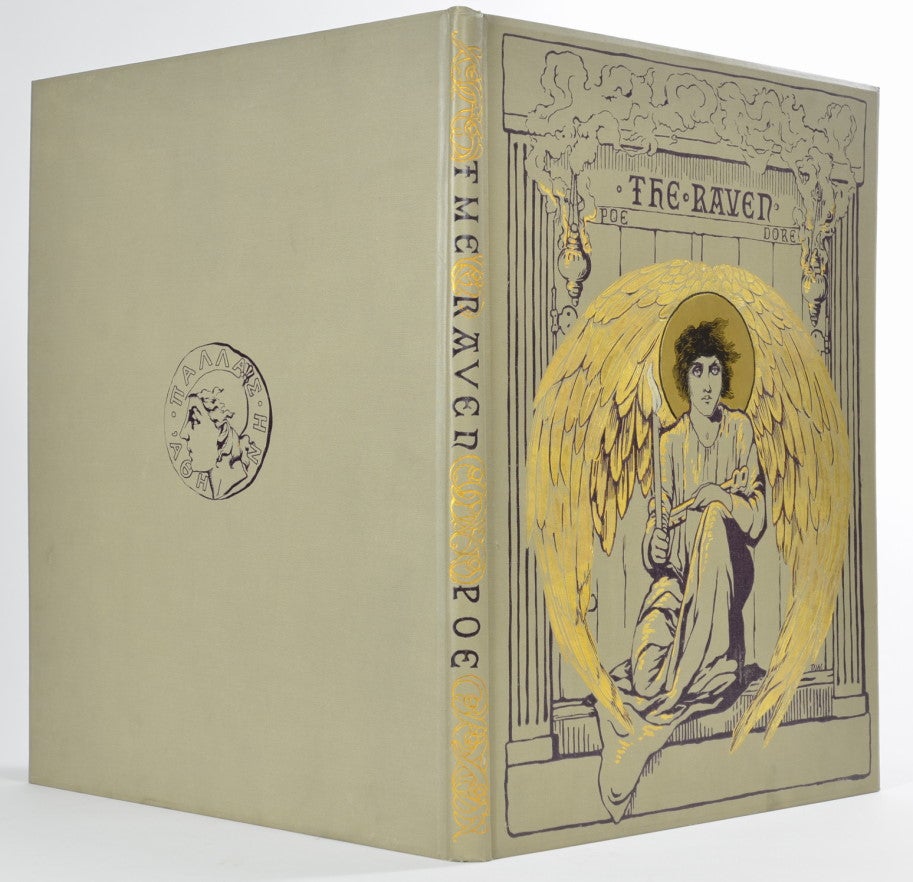The image depicts an open hard-covered vintage edition of "The Raven" by Edgar Allan Poe, likely from the 1920s. The book has a light green hardbound cover with gold leaf designs. The spine features an engraved-looking script that reads "The Raven" and "Poe." On the front cover, above the title "The Raven," is an intricate illustration of an angelic figure. The angel, donned in a long white robe that goes past its knees and over a podium, has a halo and large gold wings rendered in gold leaf. The figure is holding a candle in its right hand and a key in the other. Beneath "The Raven," the names "Poe" and "Dore" are inscribed on either side. The back cover presents a design resembling a Roman or Greek coin with uneven edges, showcasing a profile bust of a person with some Greek letters visible around the circumference. The overall coloration of the cover artwork is primarily dark grey and tan cream, except for the golden highlights.